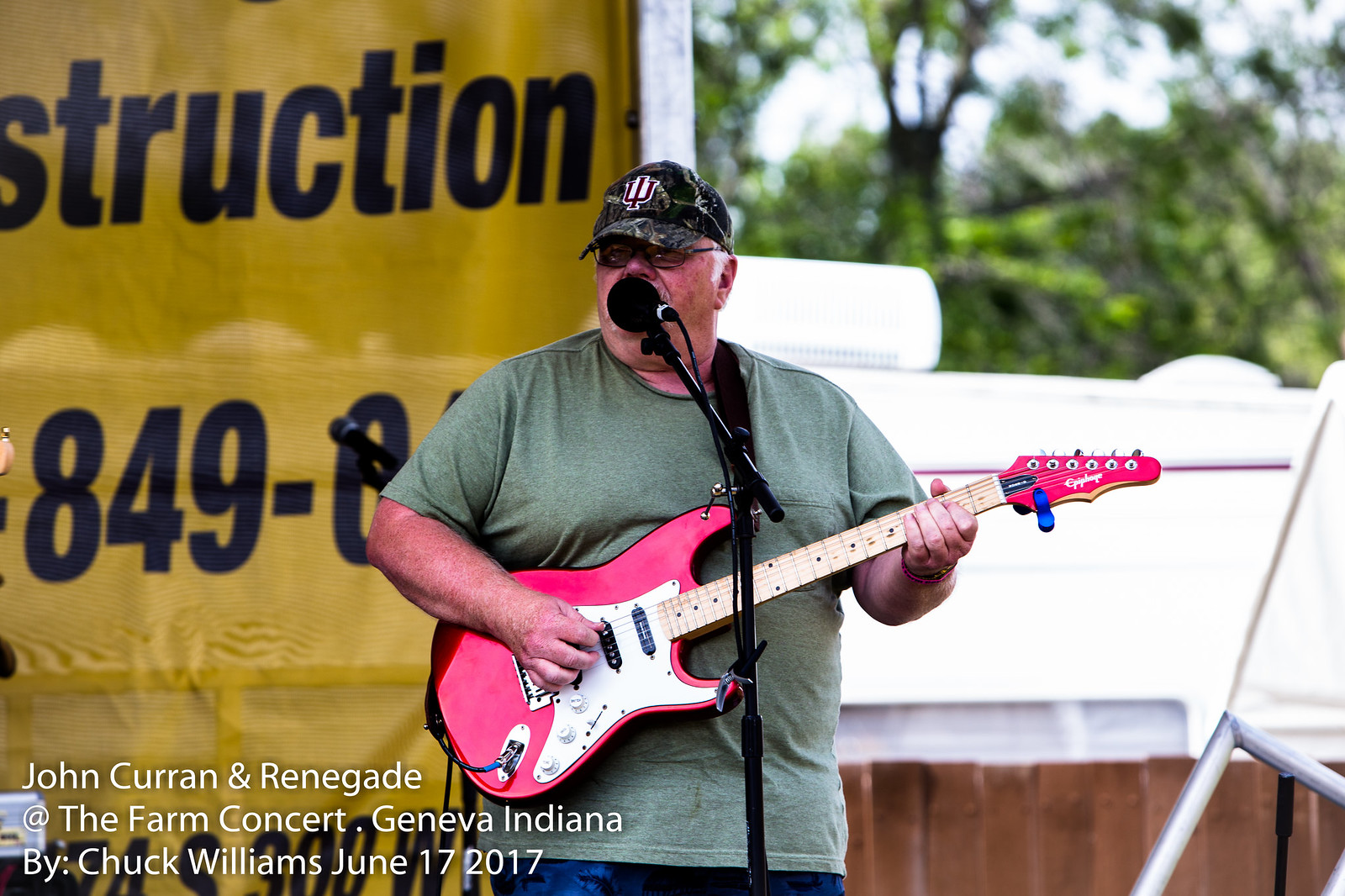The image captures a man performing on stage at an outdoor farm concert in Geneva, Indiana. He is holding an electric guitar with a unique red, white, and brown design. The man, who appears to be in his 40s or 50s, is wearing a green short-sleeved shirt, a black cap with a red logo, sunglasses, and blue jeans. He stands in front of a microphone, immersed in his performance. In the background, there's a partially obscured yellow banner with the text "Construction" and the number "849." Blurred trees and a brown fence add depth to the scene. In the bottom left corner, white text reads, "John Curran and Renegade at the Farm Concert, Geneva, Indiana, by Chuck Williams, June 17, 2017," suggesting the image was likely taken by a fan during this casual outdoor event.